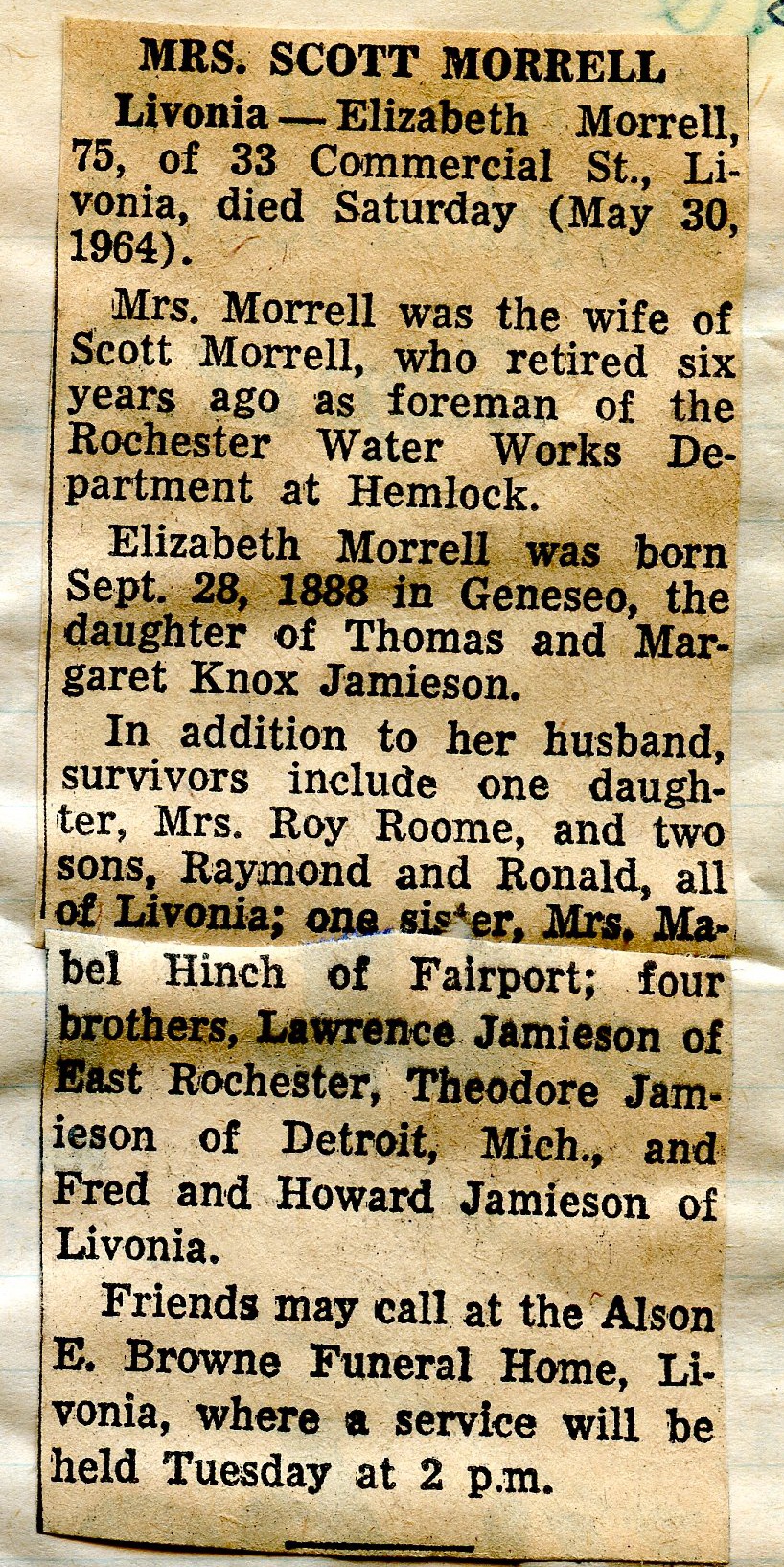This image depicts a sepia-toned snippet of a newspaper clipping, prominently centered and taking up most of the frame, set against a sheet of notebook paper. The headline reads "Mrs. Scott Morrell," and the text provides an obituary for Livonia Elizabeth Morrell, aged 75, residing at 33 Commercial Street, Livonia. She passed away on Saturday, May 30th, 1964. Elizabeth was the wife of Scott Morrell, who retired six years prior as a foreman at the Rochester Water Works Department in Hemlock. Born on September 28th, 1888, in Geneseo, Elizabeth was the daughter of Thomas and Margaret Knox Jameson. She is survived by her husband Scott, one daughter, Mrs. Roy Rome, and two sons, Raymond and Ronald, all of Livonia. Additionally, she is survived by one sister, Mrs. Marbel Hinch of Fairport, and four brothers: Lawrence Jameson of East Rochester, Theodore Jameson of Detroit, Michigan, and Fred and Howard Jameson, both of Livonia. Friends are invited to call at the Allison E. Brown Funeral Home in Livonia, where a service will be held on Tuesday at 2 p.m. The predominant colors in the image are tan, brown, black, white, and light blue.